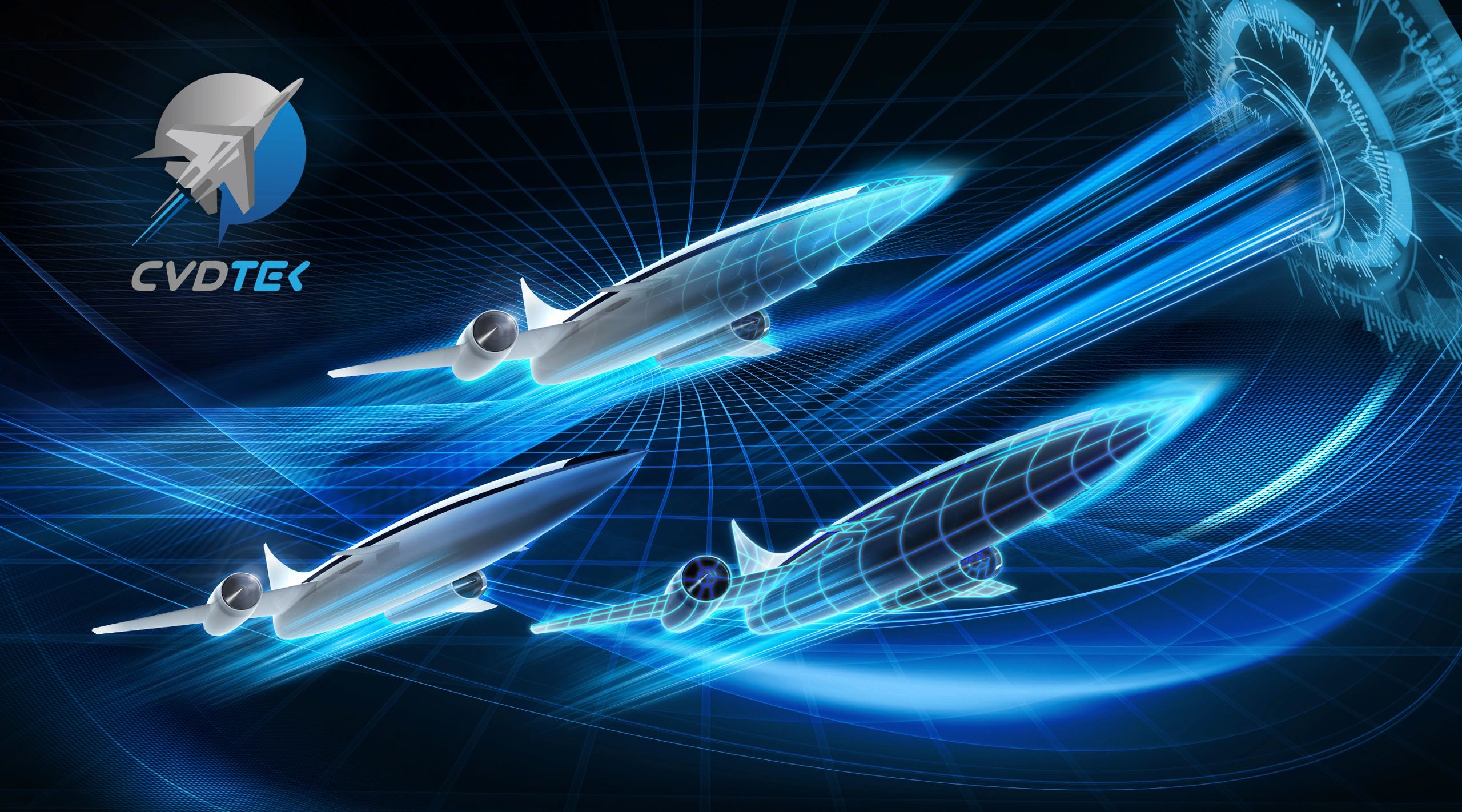The image presents a futuristic digital scene with a predominantly black and dark blue background intertwined with a sci-fi styled vortex grid pattern. In the upper-left corner, there is a prominently displayed logo labeled "CVDTEK," marked by an elegant design in shades of gray and blue. Below the logo, a series of flying crafts, resembling a mixture of fighter jets and rocket ships, are vividly depicted. There are four of these crafts, varying in size and each emanating a striking blue aura. These ships are spaced in such a way that they appear to be launching or flying from left to right across the image, with trailing blue beams accentuating their motion. The combination of the digital vortex effect and the dynamic positioning of the crafts gives the scene an energetic and high-tech atmosphere.